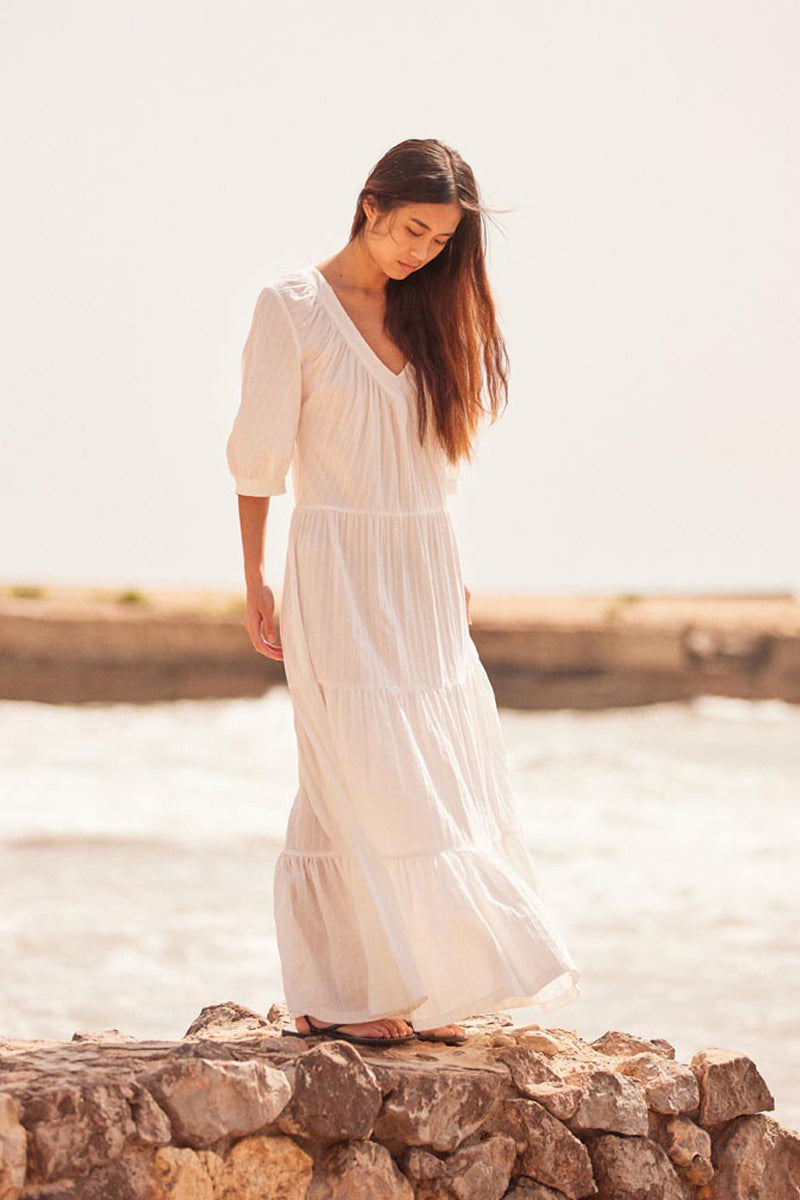In this evocative photograph, a young woman, likely in her late teens or early twenties, stands pensively on a rough, pieced-together stone wall by the water. She has long brown hair cascading over her left shoulder, with strands gently lifted by a light breeze. Dressed in a flowing, partially see-through white gown with a V-neck and short sleeves, she gazes downward, her attention focused on the rocky surface beneath her sandaled feet. The gown's ethereal quality is complemented by the simplicity of her sandals, which appear to be either brown or black. Behind her, the background remains softly blurred, revealing indistinct rolling water and an enigmatic rocky cliffscape under a gray, cloudy sky, contributing to the image's introspective mood.